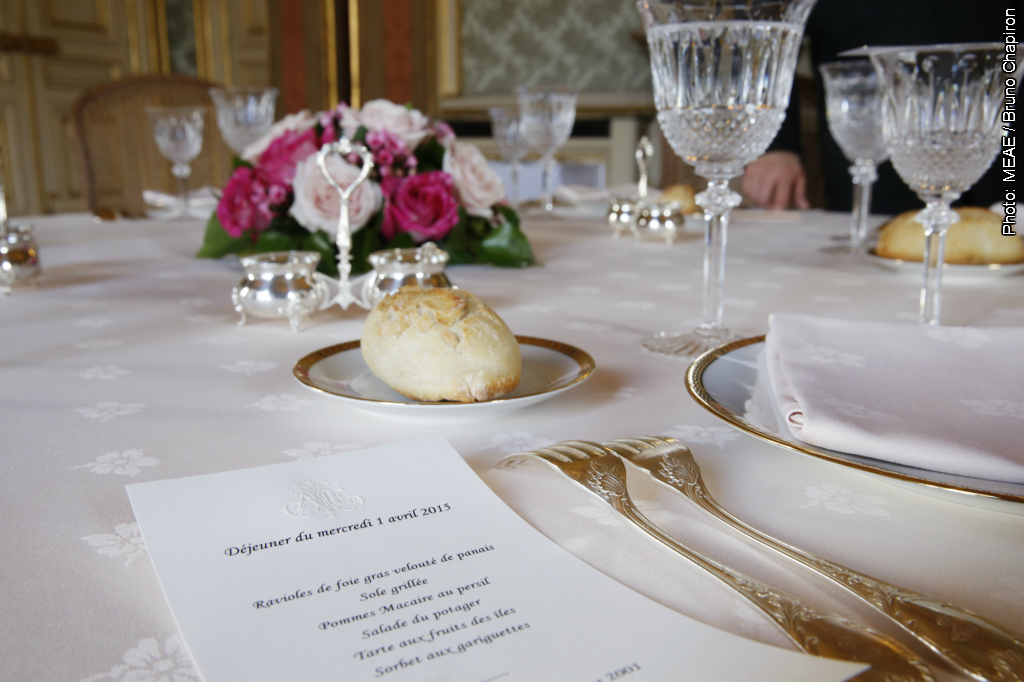This image portrays an elegantly set dining table, likely within a grand ballroom or high-end dining room. The table is adorned with a white tablecloth featuring a delicate white floral print. At each place setting, there's white porcelain china trimmed with intricate golden designs, accompanied by two silver forks and crystal-clear glasses, contributing to the refined atmosphere. Each place also includes a smaller plate with a golden rim, each holding a single roll. A thick, white menu card with French text, mentioning items like salad, sorbet, and ravioli, lies at the bottom left of the picture. It's dated April 2015 and features dishes like Tartar and Oxfruits. The centerpiece of the table includes a bouquet of flowers, adding to the table's decorative elegance. In the background, there are touches of ornate china and wood detail, while one wall is covered in wallpaper. A hand on the far right indicates the presence of a guest seated at the table.